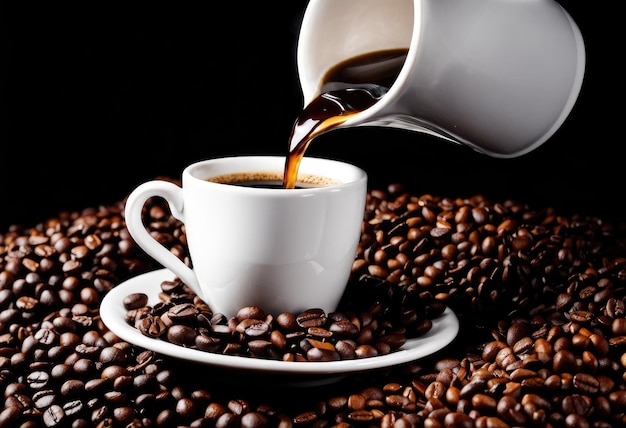In a striking landscape-format image, a pristine white ceramic coffee cup brimming with dark coffee sits on a similarly white, glossy plate. The cup rests on a substantial pile of rich, brown coffee beans, with additional beans artfully scattered across the plate. From above, a sleek white ceramic pitcher, devoid of any visible hand, pours a smooth stream of coffee into the nearly full cup. The background is entirely black, enhancing the contrast and making the whites of the cup, plate, and pitcher appear even more vibrant while drawing attention to the sumptuous coffee and abundant beans. The overall composition presents a visually captivating scene that emphasizes the elegance of the coffee-serving set against the rusticity of the beans.